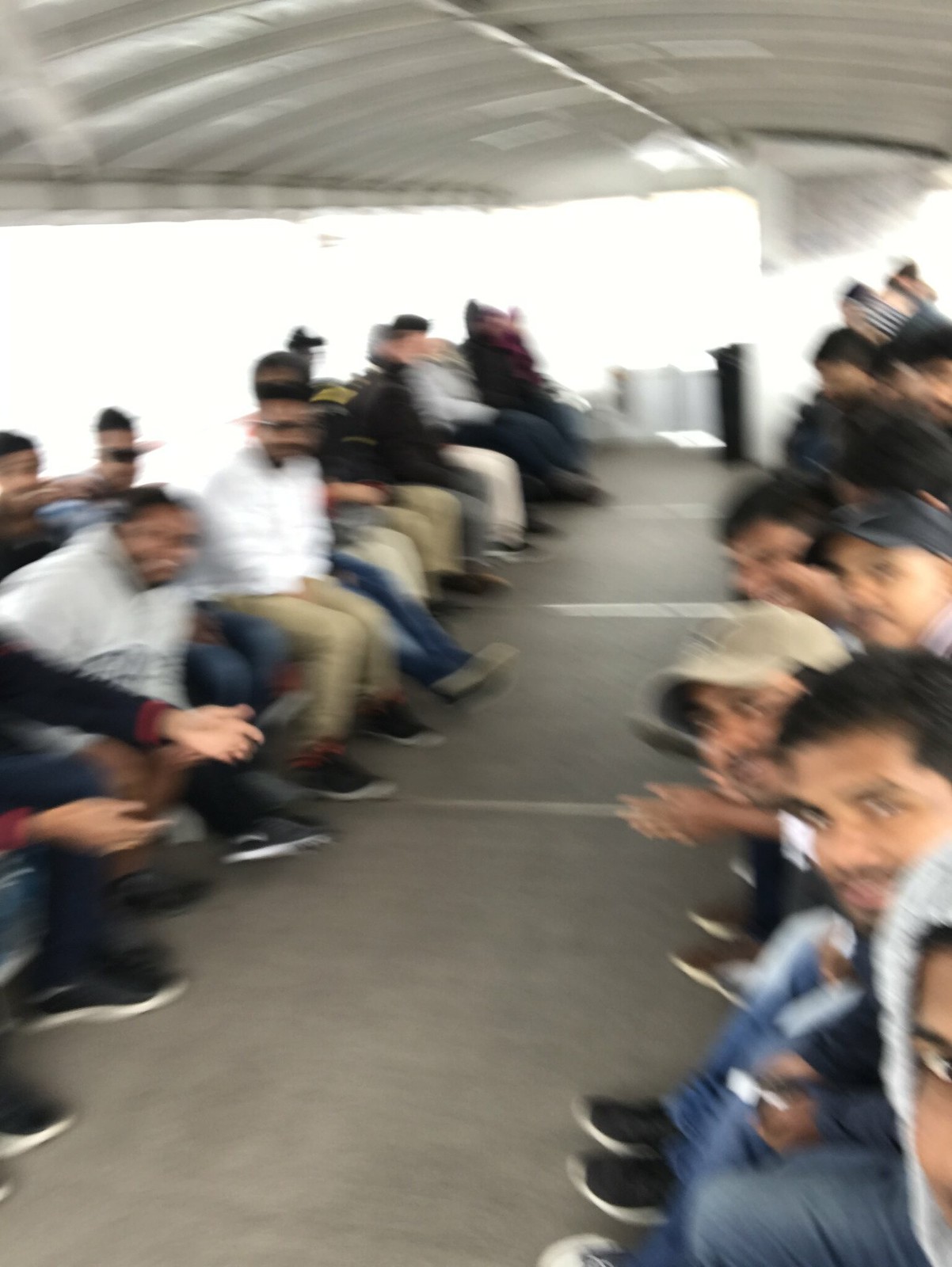A blurry image captures a group of men seated inside what appears to be a tour boat. The top of the image showcases a white arched roof, possibly made of metal. Across the roof from left to center and then to the right, there are large windows through which bright white light pours in, adding to the image's overall blurriness. 

On the left side of the image, several men are seated on a bench. Although their faces are indistinct due to the blur, it is evident that many of them are leaning slightly forward and looking towards the camera. They are dressed in a mix of white, black, and tan clothing. On the right side, another bench holds more men seated in a similar fashion, stretching from the bottom to the top of the image. One younger man, seated on the lower right, is somewhat more distinguishable and is also leaning forward like those on the left. 

An intriguing detail is that all the men appear to be wearing identical shoes—black tops with white soles.